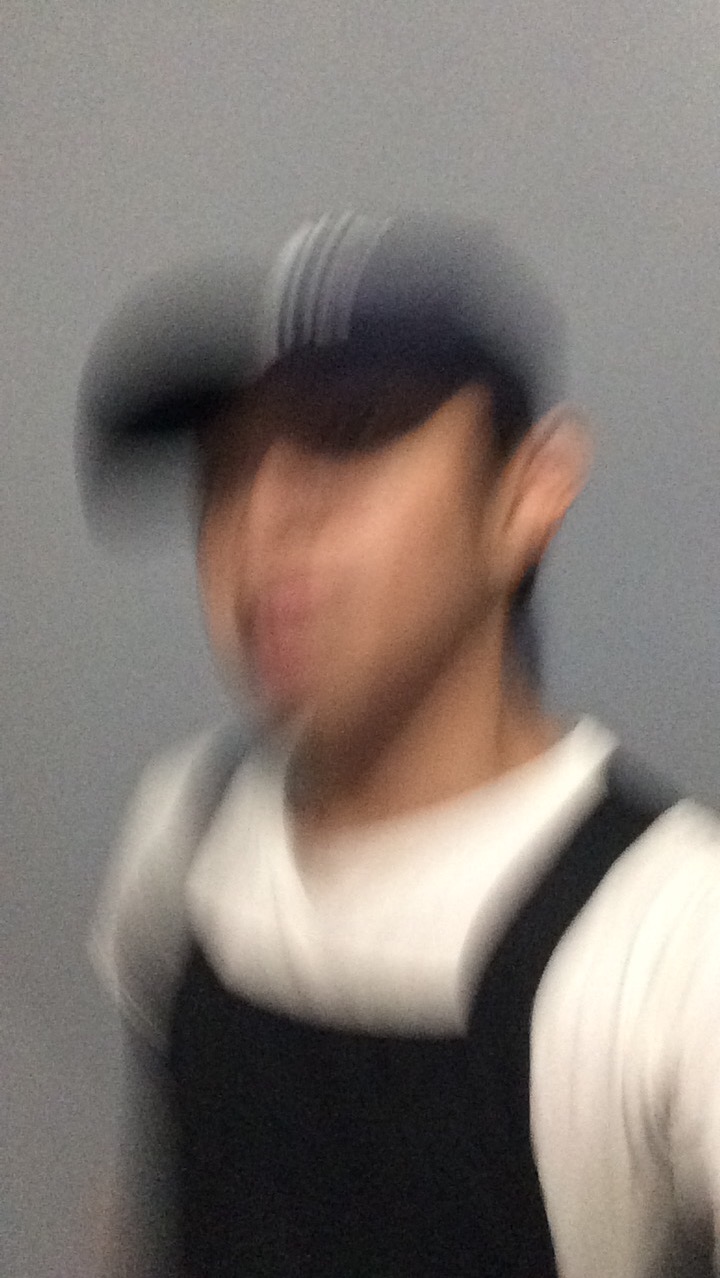"Portrait of an individual, rendered with a captivating motion blur effect that introduces a dynamic sense of movement. The subject's features are deliberately kept indistinct, emphasizing the fluidity of motion over precise detail. Clad in a sleeveless white shirt, layered beneath practical black overalls, and topped with a casual baseball cap, the person's attire suggests a blend of comfort and functionality. The setting is minimalistic, likely indoors with a plain, unobtrusive backdrop that further accentuates the motion-centric composition. This abstract approach shifts focus from clear characterization to the ethereal essence of motion, creating a visually intriguing and evocative image."